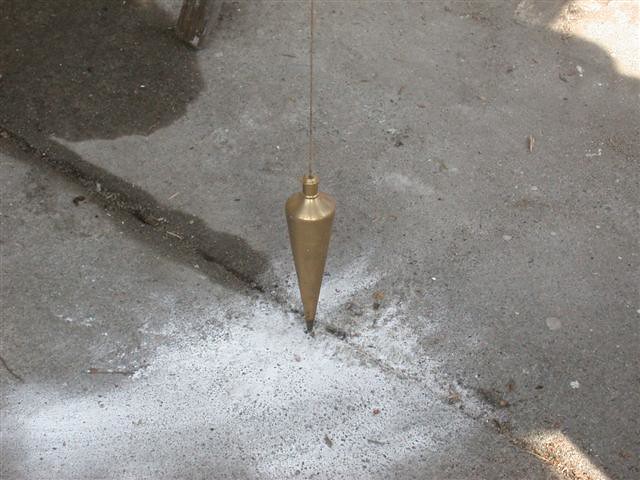In the daylight, an old-school plumb bob with a string and cone-shaped, gold attachment dangles over a weathered concrete sidewalk. The pointed tip of the plumb bob hovers near the surface, which features chalk markings and white discolorations. Shadows cover most of the image, with sunlight highlighting the top right and bottom right corners. The top left corner appears wet, likely from a liquid spill, and there are sticks and debris scattered across the sidewalk. Additionally, a part of a wooden post is visible, adding to the scene's rustic ambiance.